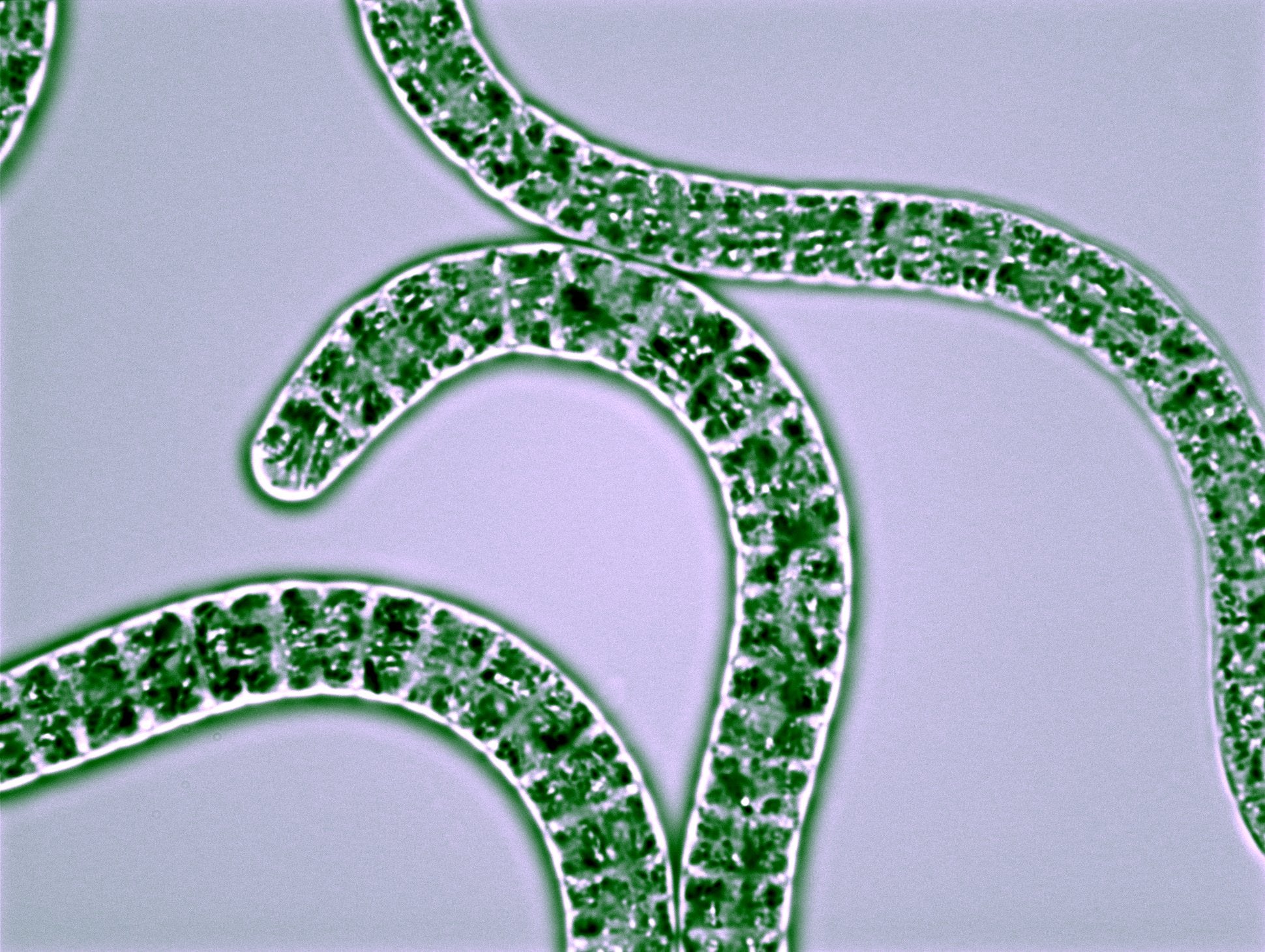The image depicts a microscopic view of possibly worm-like organisms or bacteria against a light gray to lavender background. Several elongated, snake-like figures are scattered across the scene. These figures are predominantly green with dark green parts and are outlined by white borders. Their interiors feature splotches of various shades of green and occasionally white. The shapes are serpentine, winding across the field, with some touching or intersecting each other. The largest one arcs across the image, curving down the right side, while others form intricate shapes like question marks, contributing to a complex, interwoven pattern. The background is clean, highlighting the detailed, textured organisms against it.